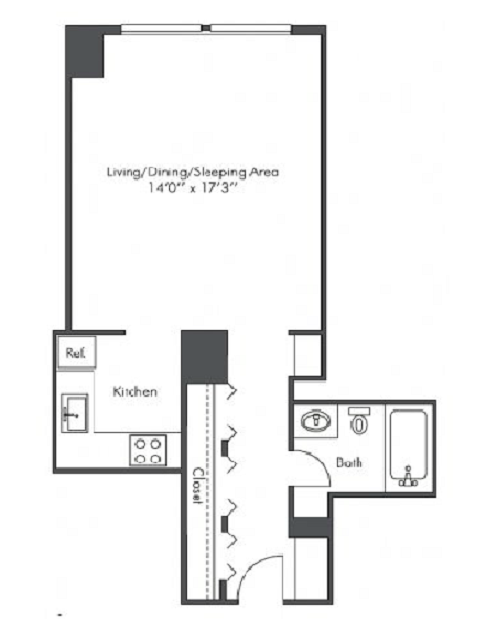This floor plan depicts a cozy studio apartment, characterized by a single, multi-functional main area measuring 14 feet by 17 feet 3 inches. This central space, labelled as the living, dining, and sleeping area, features two windows positioned at the top, providing natural light. The layout offers two possible directions upon exiting this primary room.

To the left, you enter a compact kitchen equipped with essential amenities: a stove top, refrigerator, and sink, but notably lacking a dishwasher and pantry, underscoring the efficient use of space.

Alternatively, heading downward from the main area leads into a corridor. On the right side of this hallway, there is a small closet followed by a compact bathroom containing a sink, toilet, and bathtub, with an additional small closet possibly located within the bathroom itself. Continuing down the corridor, a series of closets with folding doors line the left side, offering ample storage. The hallway ultimately leads to the apartment entrance.

This layout suggests a typical New York-style apartment, inferred from the limited window placement, confined to the main living area, maximizing the use of available space within the urban setting.